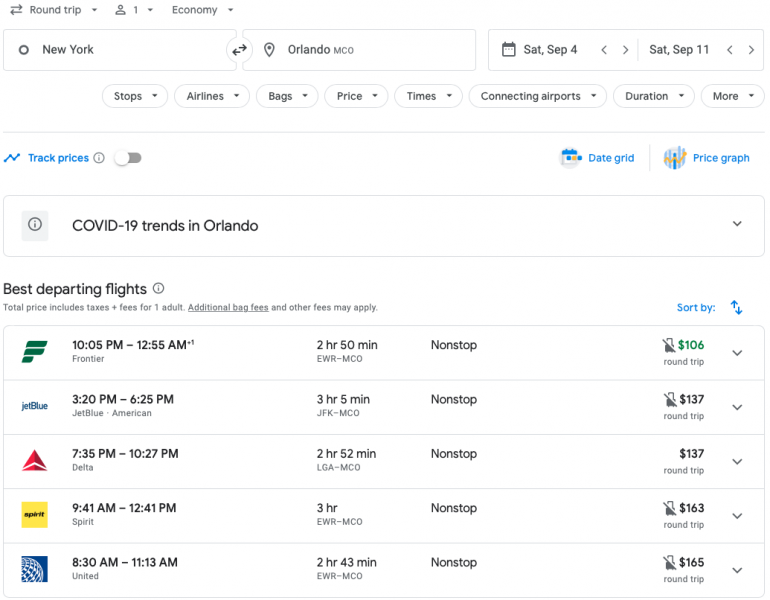The depicted image is of a flight booking website. The top left corner features navigation options for a roundtrip, with drop-down menus for the number of passengers (set to one) and the class of service (Economy). The flight route is specified from New York (NYC) to Orlando (MCO), with text fields to input the travel dates, currently set from Saturday, September 4 to Saturday, September 11. 

Below these options, there are several buttons with drop-down menus for refining the search, including "Stops," "Airlines," "Bags," "Price," "Times," "Connecting Airports," "Duration," and "More." There is also an option to "Track Prices" via a toggle switch, which is currently off and highlighted in blue. To the right, there are additional resources such as a "Date Grid" and a "Price Graph," both also in blue.

Further down, there is a section for COVID-19 trends in Orlando, with a drop-down menu on the right for additional information. The website lists the best departing flights, with the total price including taxes and fees for one adult. Note that additional baggage and other fees may apply. 

Featured flights include:
- Frontier: Departing at 10:05 PM and arriving at 12:55 AM, with a non-stop 2.5-hour flight from EWR to MCO, priced at $106 round-trip.
- JetBlue: Departing at 3:20 PM and arriving at 6:25 PM.
- American Airlines: With a flight duration of 3 hours and 5 minutes.

The detailed layout and various options are clearly aimed at providing users with a comprehensive and customizable flight search experience.